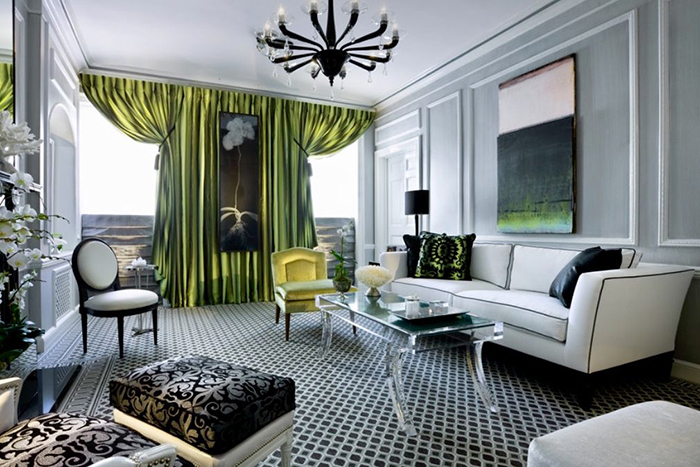This image captures a meticulously decorated and upscale formal living room with a light gray wall backdrop featuring insets outlined in white-painted wood. The room is brightened by dramatic, tall, floor-to-ceiling green or citron curtains that frame two large windows, with a prominent, rectangular painting of a single flower with white leaves hanging in the middle of the curtains. The black and white checkered diagonal patterned floor adds a striking contrast. 

Furnishings include a white couch with black stitching, adorned with black and white pillows, accompanied by a glass coffee table displaying decorative items that cohesively blend with the room's palette. Seating options feature a black and white chair with a print, a smaller plain black and white chair, and a luxurious citron-colored velour chair. The room also holds a distinctive dark gold chandelier, fashioned like an inverted octopus with light fixtures on the tips of each arm, adding an elegant yet whimsical touch. 

Additional decor elements include pictures and a painting on the walls, lampshades, flowers, and various ornamental objects strategically placed throughout the room to amplify its sophisticated and coordinated aesthetic.